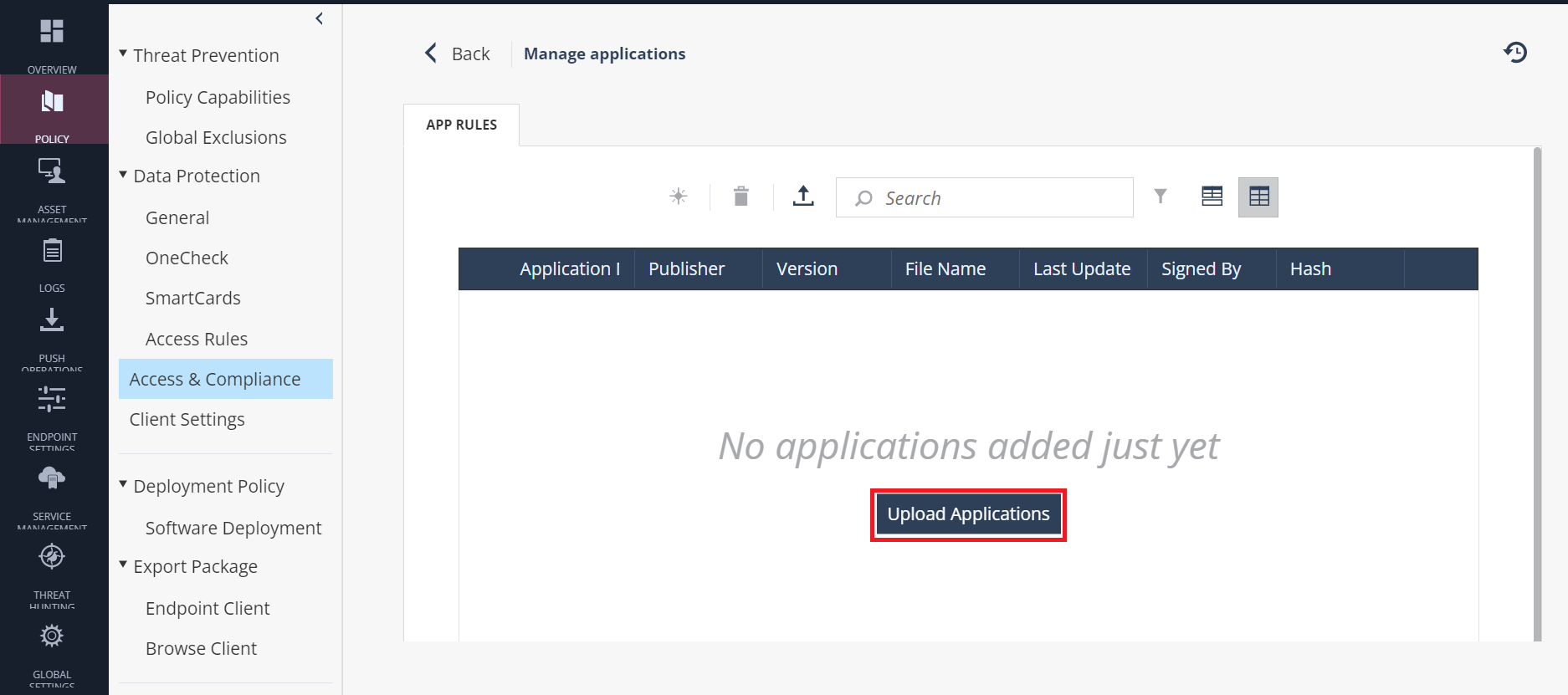This is a detailed cropped view of a screenshot showcasing firewall information. The screenshot features a predominant gray background with a very thin black bar on the left side listing various categories vertically. On the right, there is a gray column also listing categories vertically.

Under the "Data Protection" section, the "Accessing the Compliance" option is selected. An open panel to the right displays the title "Manage Applications" at the top, with a "Back" button accompanied by a left-pointing arrow to the left of it. Below this, there is a tab labeled "Open" with "App Rules" written at the top of the tab.

At the top center of the view, there is a search bar flanked by several icons: a star icon, a trash icon, a share icon on the left, and layout icons on the right. Directly below these icons runs a blue bar with categories labeled "Application," "Publisher," "Version," "File Name," "Last Update," "Signed By," and "Hash."

Towards the bottom of the screen, the text "No applications added just yet" appears in light gray. Below this message, there is a prominent blue button labeled "Upload Applications," which is outlined by a red box added to the photo.